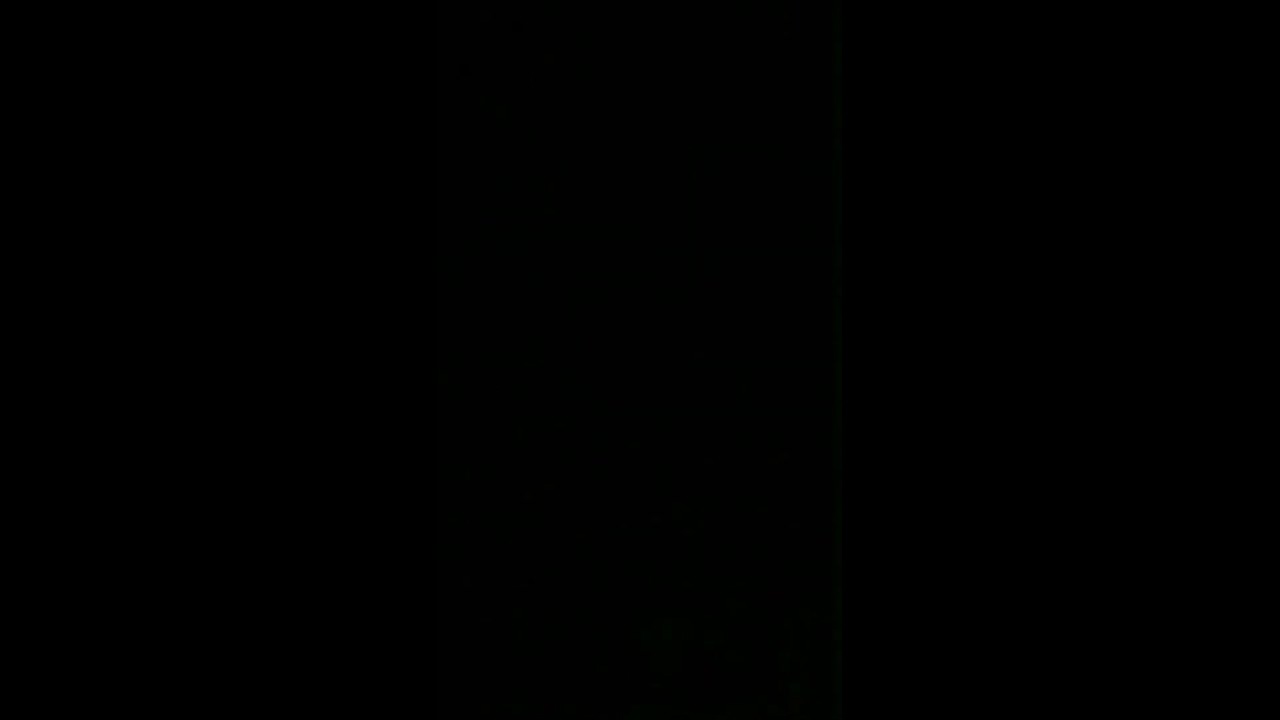The image is a perfect, plain black rectangle, measuring approximately 5 inches in length and 8 inches in width, featuring four right angles at each corner. It is completely devoid of any images, text, or additional elements, making it a solid black background. This stark, fully black rectangle could be used as a wallpaper for desktop computers or phones, or potentially signify a loading screen for a video—whether at the start or end. The pervasive darkness of the image dominates its entirely minimalistic design.